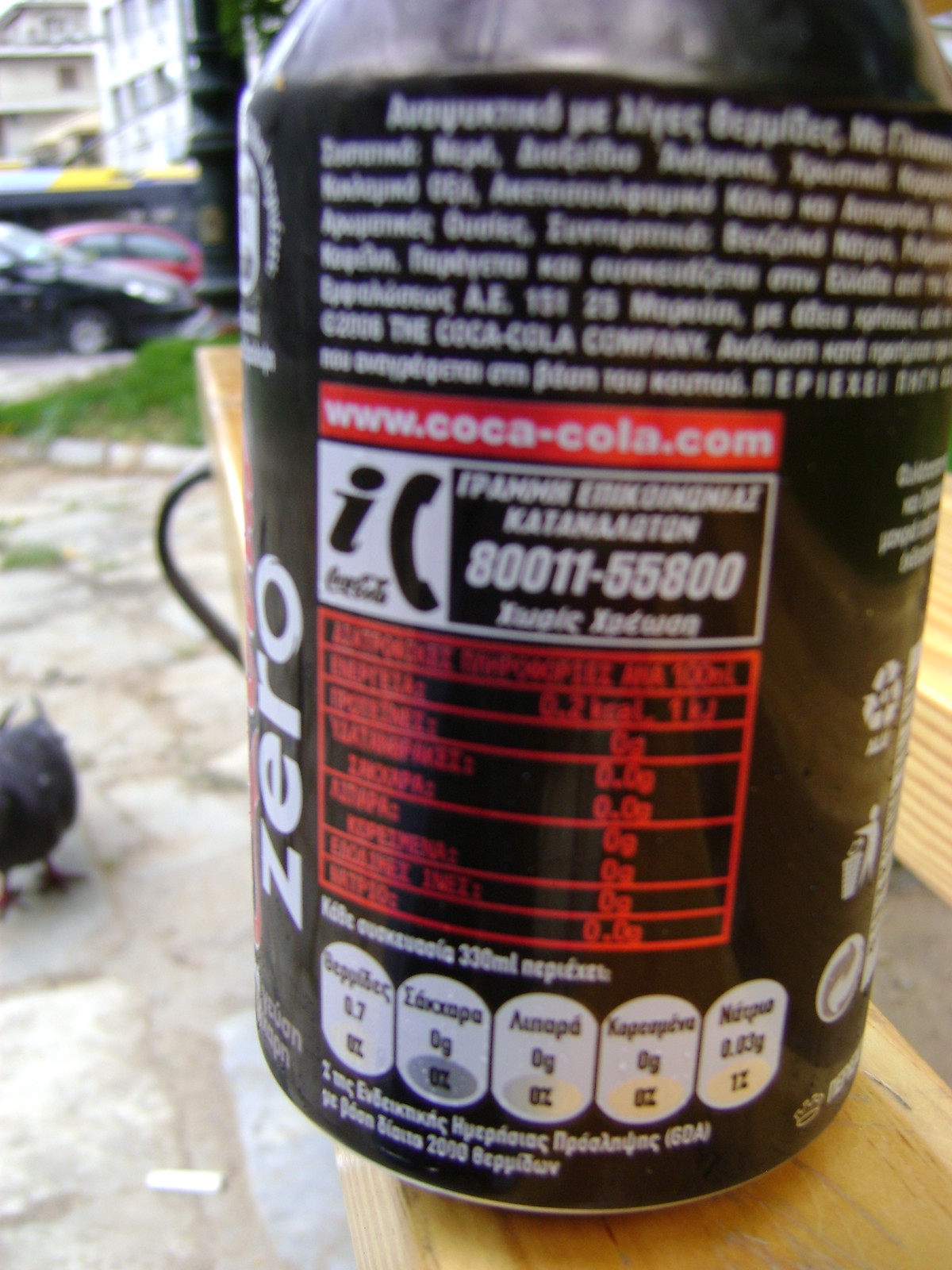A photograph of a Coke Zero can with a black label, captured from the backside. The top of the label features six lines of white text, although it's blurred and unreadable. Beneath the text, there is a web address "Coca-Cola.com" prominently displayed in a red box. Directly underneath the web address, there's a telephone number accompanied by a small phone icon. Further down, a Nutrition Facts box stands out, uniquely printed in red. Below the Nutrition Facts, five oblong shapes are lined up, each containing foreign language text and gram amounts. The can is placed on a wooden plank, and the setting is outdoors. In the background, there is a parking lot, an apartment complex, and a pigeon pecking on the ground.